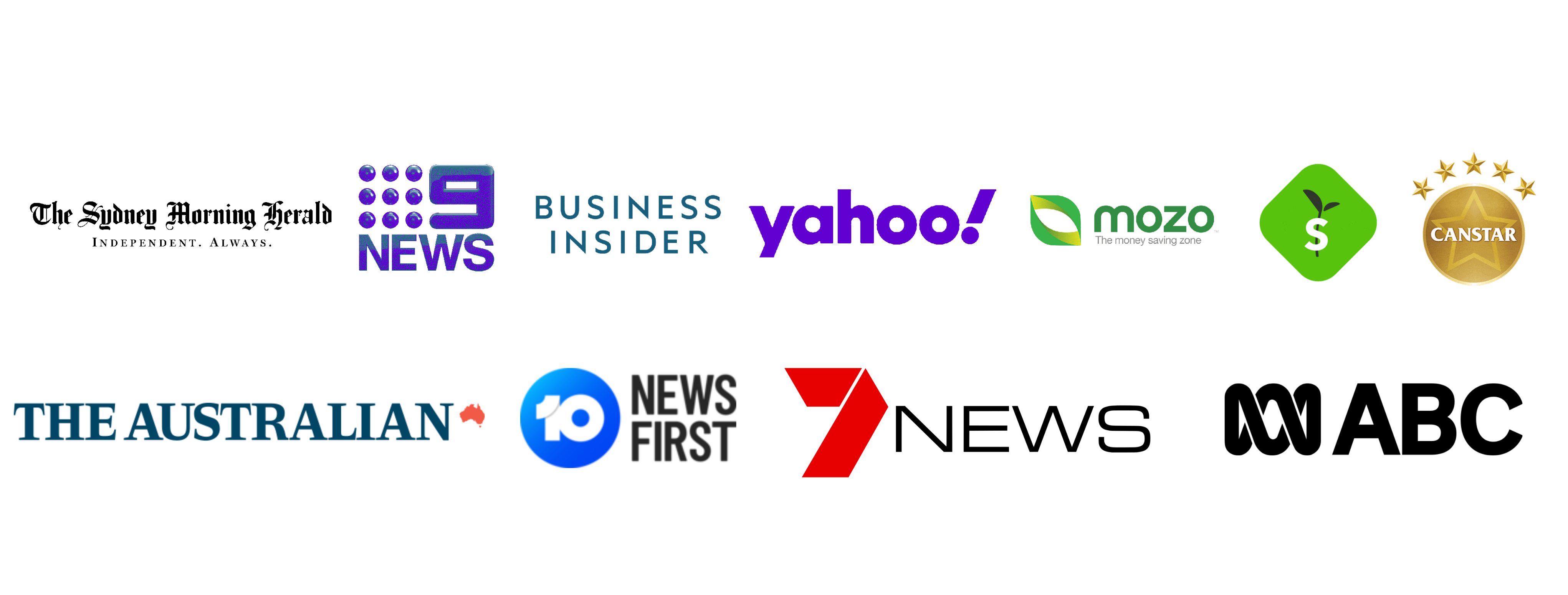This image appears to be a section from the bottom of a website that showcases various company logos, giving an endorsement effect that the product featured on the website is credible and trusted by known entities. The image is approximately five times as wide as it is tall, with a white background that seamlessly merges into the page without any defined edges.

The layout consists of two rows of logos: the first row contains seven logos while the second row has four. Here's a detailed breakdown of the logos and text positions:

1. **The Symphony Morning Herald**: Presented in black text with a traditional, newspaper-style font at the top left. Below the name, it says "independent always" in smaller text.
2. **Interpretable Graphic Representation**: Located next to The Symphony Morning Herald, featuring a 3x3 grid of purple dots in the upper-left corner, a stylized number nine to the right, and the word "News" beneath it.
3. **Business Insider**: Placed to the right, this logo is in all capital letters with a blue-green hue.
4. **Yahoo!**: On the far right of the first row, showcasing its well-known purple logo with an exclamation point at the end.

In the second row:
1. **Mozo**: Starting from the left, the text "Mozo" is written in grass green. To the left of the text, there is a logo resembling a leaf.
2. **Green Diamond Logo**: Positioned next to Mozo, this consists of a green diamond with a white S centered inside it, backed by a dark-colored plant graphic.
3. **CanStar**: Located at the far right, this logo features a gold star with the word "CanStar" in white at the center and five smaller gold stars arched above it.

These logos are representative of widely recognized entities, enhancing the credibility of the product by displaying a diverse array of endorsements from trusted sources.